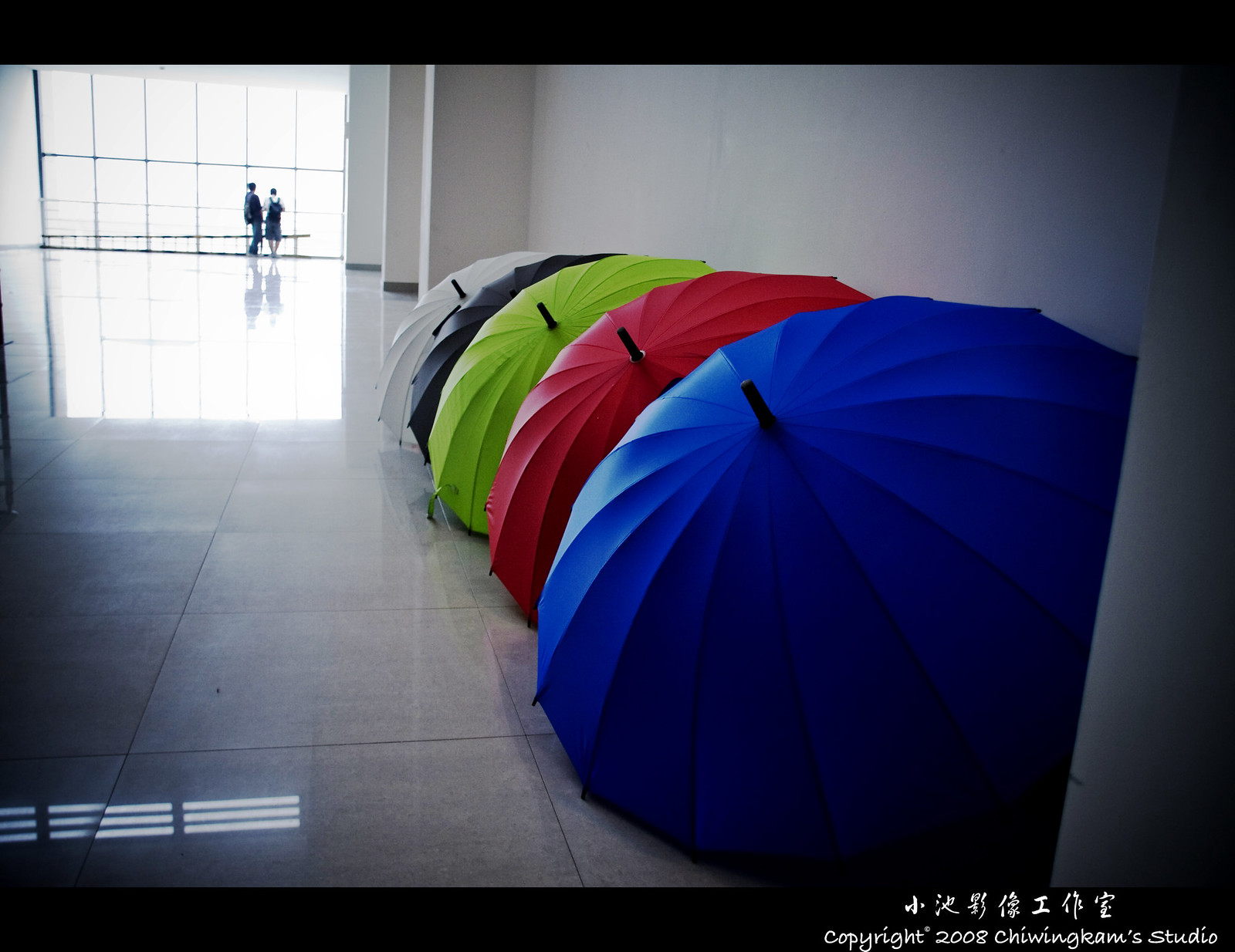This photograph captures a spacious, modern interior with a highly reflective, polished stone floor, possibly marble, extending across the area. The setting appears to be a massive, open building with floor-to-ceiling glass windows on the far wall, spanning about 15 feet high, allowing natural light to flood in and reflect beautifully off the floor. Two figures with backpacks stand silhouetted against the windows, gazing outwards.

The dominant feature of the image is a series of five vibrant open umbrellas arranged purposefully along the lower right wall of the space. From front to back, the umbrellas are royal blue, bright red, lime green, jet black, and white. Each is positioned so that the top peak is visible, aligned in a neat sequence, lending an artistic flair to the composition.

The photo predominantly features monochromatic tones of gray, black, and white, with the colorful umbrellas standing out vividly. In the bottom right corner, white script against a black border features Asian characters, accompanied by the text "Copyright 2008 Xi Wing Cam Studio." The setting, possibly resembling an airport or a vast lobby, is meticulously clean with sleek lines and a serene, almost minimalist atmosphere, underscoring the striking visual impact of the umbrellas.